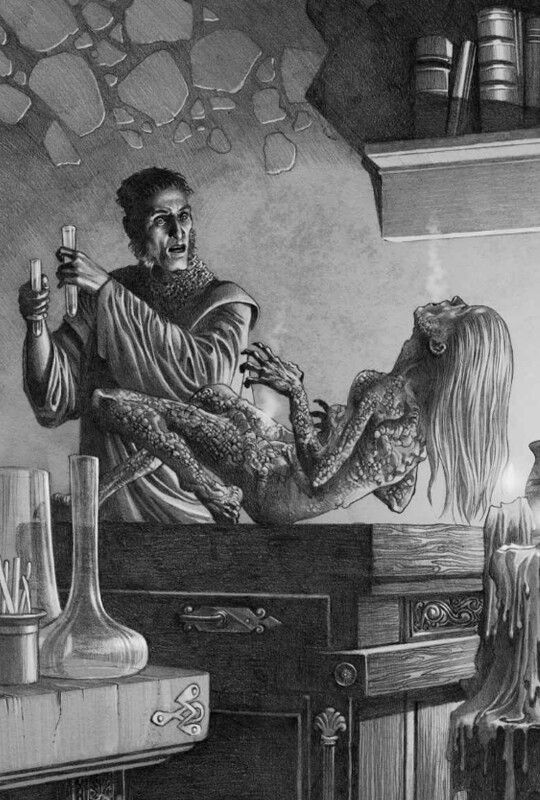The image is a detailed black-and-white drawing depicting a mad scientist in the midst of a disturbing experiment on a woman who is laying on a wooden table. The woman appears to be in extreme agony, her body covered in severe burns as the scientist pours chemicals onto her. She is partially rising off the table, her long hair cascading down while her head is lifted in pain. The scientist, who has short brown-black hair and long sideburns, wears a long cloak and has a shocked expression on his face as he witnesses the horrific effects of his experiment.

The background features a stone wall at the top and a bookshelf to the right, filled with thick, ancient-looking books. The wooden table the woman is on is intricately detailed, showing the grain of the wood and metallic elements. To the right of the scene, there are melted candles, while to the left, another table holds several rounded-bottom flasks, emphasizing the laboratory setting of this grim scene.